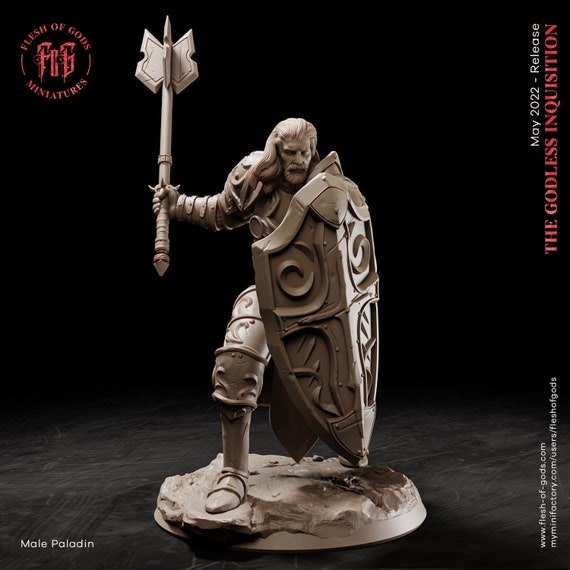This image features a detailed, unpainted figurine of a fierce warrior, resembling an old-school paladin or Viking. The figure, sculpted out of a beige-gray clay or a similar material, stands on a rock-like base against a black background. The warrior has long, flowing black hair cascading down his shoulders and a full beard, exuding a menacing and battle-ready demeanor. He is adorned in partial knight's armor on his legs, arm, and chest. In his right hand, he wields a massive, intricate weapon that resembles a combination of a spiked mace and a four-sided axe, poised for a swing. His left hand bears a large, heavy shield, almost as tall as the figure itself, featuring an ornate top and a cross insignia. 

Text elements frame the image: on the top left, a circular red logo reads "Flesh of God's Miniatures," while the bottom left features "Male Paladin" in red and white text. The top right indicates the release date as "May 2022 Release," with the additional title "The Godless Inquisition" in red text below it. URLs are listed on the bottom right, including "www.flesh-of-gods.com" and "www.myminifactory.com/user-fleshgods." Voila, a striking and intricately detailed warrior sculpture ready for release in May 2022.